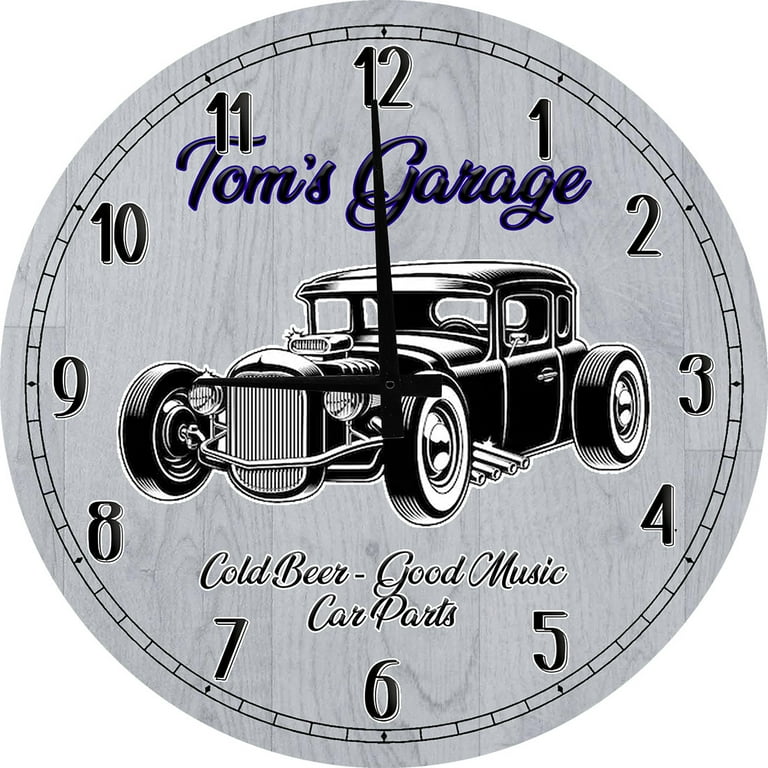The image features an old-fashioned gray wall clock with a wooden texture, showcasing an advertisement for Tom's Garage. The clock itself displays the time at 9 o'clock, with black numbers and black hands. At the top of the clock face, there is a cursive script in dark blue or purple that reads "Tom's Garage." Below this, a black-and-white depiction of an early 20th-century roadster, possibly a Model T or one of its successors, is centrally positioned. Further down in smaller cursive script, it reads "Cold Beer, Good Music, Car Parts," hinting with a touch of irony that the clock might be advertising a vintage-themed bar created from a converted garage. The overall aesthetic of the clock is simple yet charming with its muted colors of gray, black, and blue.